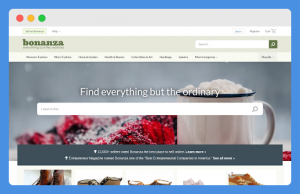This image is a detailed screenshot of a website's homepage, displayed within a blue border. The top part of the screenshot features a gray and white background, with a distinctive rectangular gray box on the left housing three colored buttons: red, yellow, and green. Below this, a prominent white box possibly serves as a search box, accompanied by two buttons beside it on the left. To the right within this white box are three additional buttons, among which one seems to depict a card icon, possibly related to sign-in options.

Beneath this section, a gray box spans the width, displaying the name "Bonanza" on the left side—likely indicating the website’s branding. Adjacent to this, on the right side of the gray box, is a smaller white search box. Below this, a horizontal menu bar extends almost the entire width, though the specific menu options are not fully readable.

Further down, a central photo appears, possibly depicting a mug with coffee or another solid substance. Overlaid text on this image reads "find everything but the ordinary," alongside another search box and a gray box with additional text. The screenshot concludes with partial views of additional images at the bottom, not wholly visible.